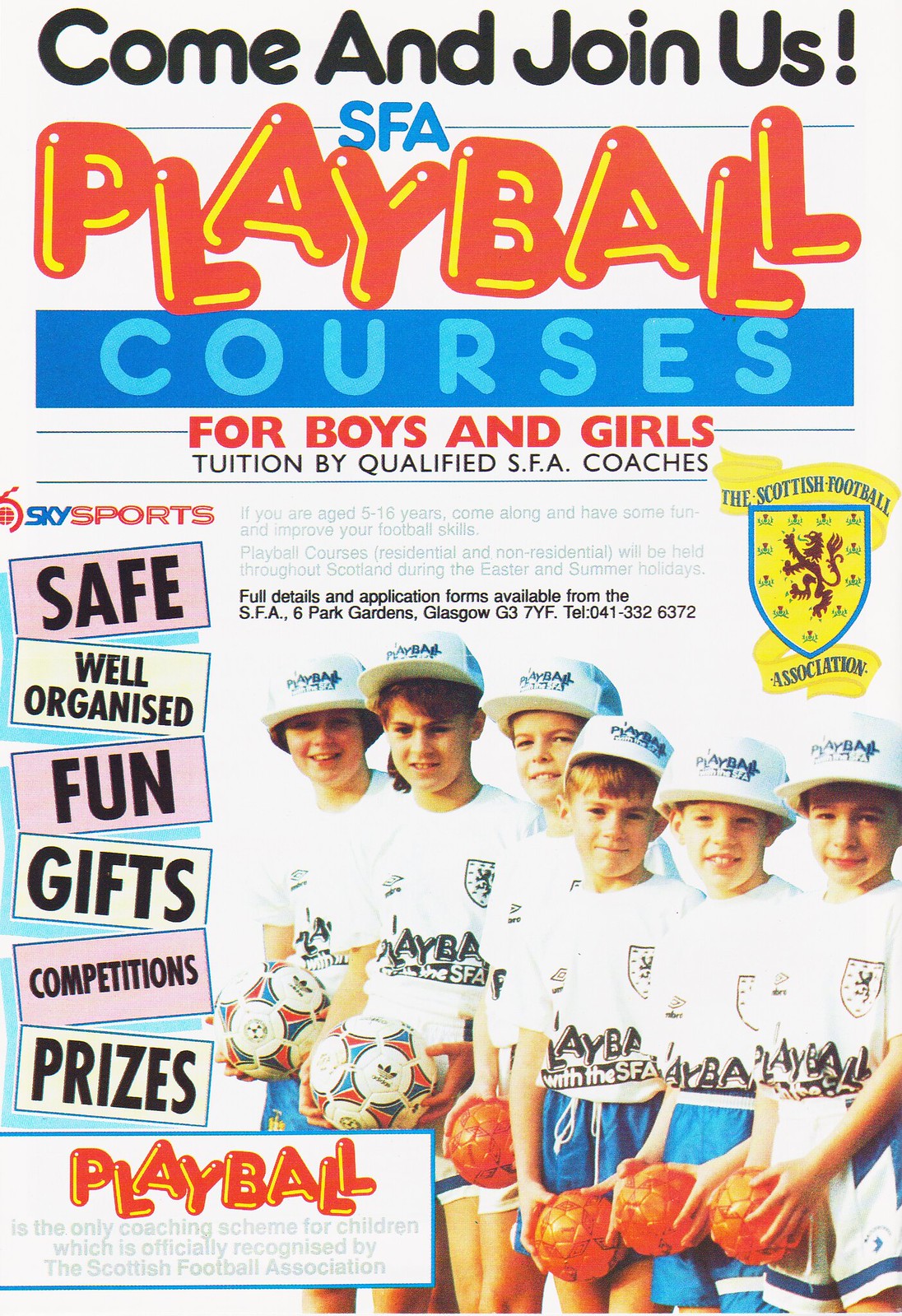The image is a color-printed flyer in portrait orientation, with a creamy white background promoting a youth team event. At the top, bold black letters announce, "Come and Join Us!" followed by "SFA" in blue text. The main highlight, "Play Ball," is displayed in playful, bubbly red letters with yellow lines inside. Below this, a blue box contains the word "Courses," followed by red lettering that states, "For Boys and Girls." Further down, black text declares, "Tuition by Qualified SFA Coaches."

On the left side of the flyer, bullet points in various colors list the features: "Safe, Well Organized, Fun, Gifts, Competitions, Prizes." To the right of the text information, a color photograph showcases a row of five young boys, arranged from shortest to tallest, all wearing white t-shirts with "Play Ball" printed on them and white baseball hats. Some of the boys are holding small dodgeballs, while others hold larger soccer balls. All of them are smiling and appear to be in early elementary school, possibly around first grade. At the very bottom left corner of the flyer, the word "Play Ball" reappears, solidifying the playful and inviting theme of the event.